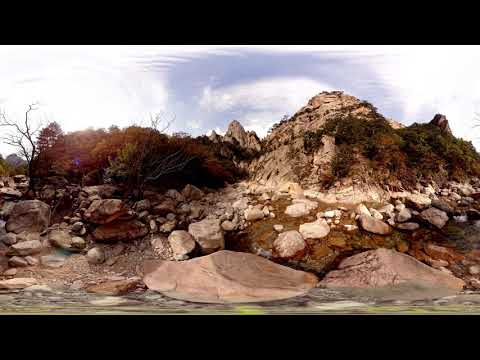This image showcases a striking landscape featuring a rugged rocky outcropping with a variety of rock formations, creating a distorted yet captivating scene. The foreground is dominated by brown boulders and smaller broken rocks scattered along a shore-like area, where there appears to be a creek or river running through. This rocky terrain gradually rises into a more prominent hill or small mountain, adding depth to the composition. 

The environment is dotted with some vegetation, including trees with both green and reddish leaves, and some that are bare. The flora is predominantly found from the left side to the center of the image, with shorter tree branches and possible presence of moss, lichen, or short grass on the rocks by the shore. 

Above this intricate landscape, the sky is a mix of white clouds and patches of blue, giving it a partly cloudy appearance with sunlight breaking through. The overall outdoor scene creates a compelling contrast between the earthy tones of the geological features and the sporadic bursts of natural greenery, set against a bright yet somewhat cloudy sky.